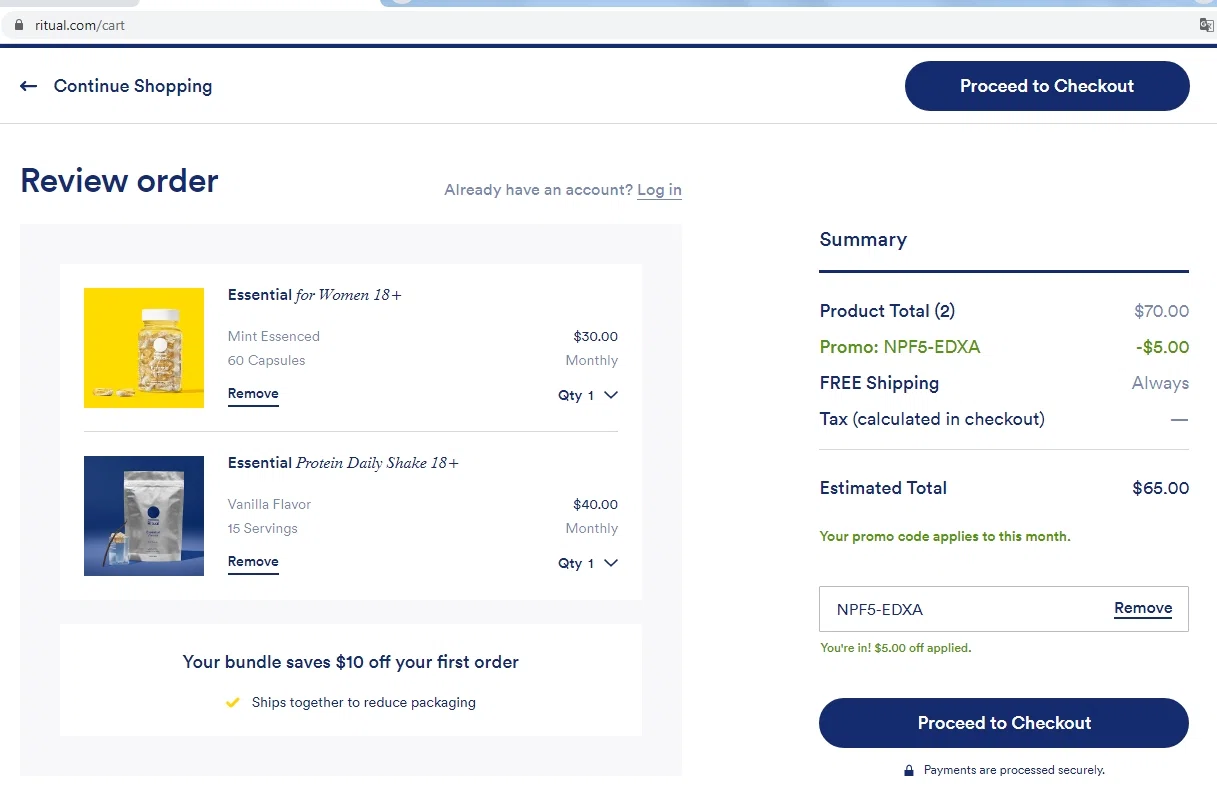This image depicts a part of the online checkout process on the website ritual.com, specifically at the URL ritual.com/cart. The top of the screen features a dark blue line dividing the webpage header from the checkout information below. 

On the left side of the header, a left-pointing arrow accompanied by the text "Continue Shopping" is displayed in blue font, allowing users to return to the product selection page. On the far right, an oblong clickable button is visible, saying "Proceed to Checkout" in white font set against a blue background.

A lighter, thinner blue line separates this header from the main content area. Immediately below this, "Review Order" is written in blue text, guiding users to the section where they can verify their selected products. In the middle of this section, a prompt asks, "Already have an account? Login", with "Login" underlined in a lighter blue font, facilitating existing customers to sign in.

The central portion of the image showcases two thumbnail images of items in the cart. The first item is "Essential for Women, 18+ Mint Essence, 60 Capsules," showing a pill bottle with vitamins. The second item is "Essential Protein Daily Shake, 18+ Vanilla Flavor, 15 Servings," depicted as a packet of protein shake mix. 

The capsule product is priced at $30 monthly with a quantity of one, while the protein shake is listed at $40 monthly, also with a quantity of one. Below these items, a promotional offer is highlighted in blue text: "Your bonus $16 off your first order, shipped together to release packaging."

On the right side of this section, an order summary is provided, segmented by blue lines. It details the product total, applied promotion, free shipping, tax, and the estimated total. A promo code has been entered in the designated box, deducting $5 from the total, and the user is ready to finalize the purchase by clicking the "Proceed to Checkout" button.